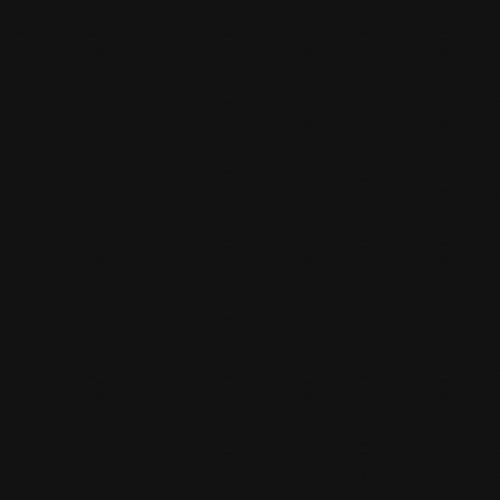This image features a completely black square, accentuated by a very subtle, thin yellow border that is almost imperceptible. The deep, uninterrupted blackness of the square evokes a sense of vast emptiness, reminiscent of a starless, moonless night sky devoid of any visual or auditory disturbances. This profound simplicity leaves much to the viewer's interpretation, conjuring various associations such as the straightforward elegance of black clothing, often considered slimming and easy to wear. Despite its minimalistic appearance, the black square invites introspection and contemplation, offering a blank canvas for the imagination.